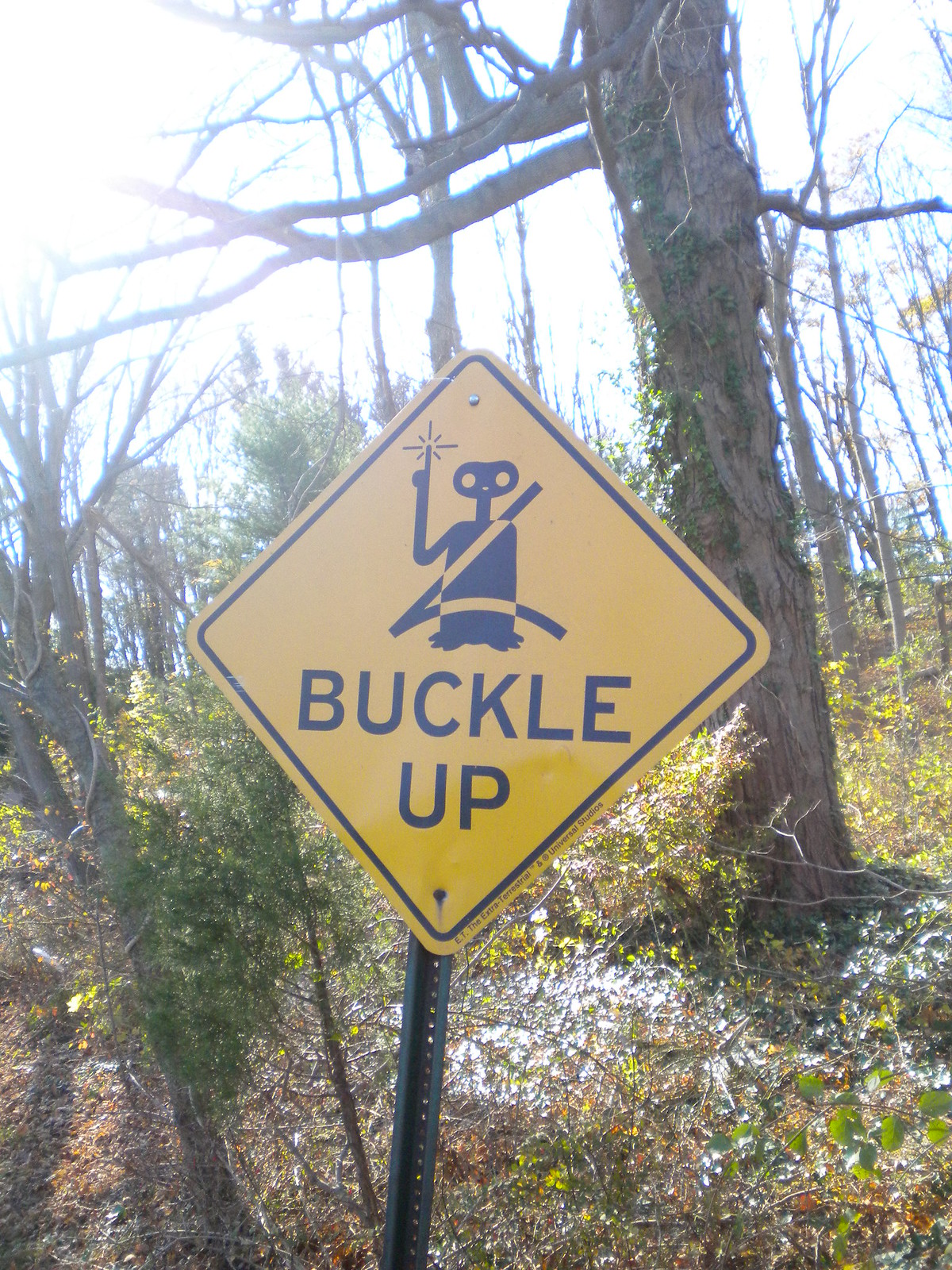The image captures a serene outdoor setting with the sky visible above, casting a radiant white glow, particularly in the top left corner. In the midground, a distinct yellow diamond-shaped sign stands out among the trees. This sign features a black border and displays a black artwork of a person wearing a seatbelt, with the strap secured over their shoulder and lap. Below the illustration, the caption "Buckle Up" is prominently written in black. Additional text is visible in the bottom right corner of the sign.